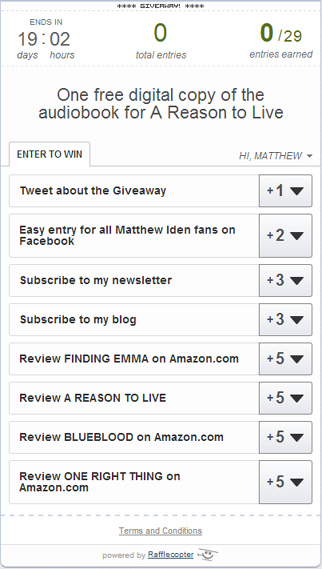### Caption:

The image showcases a webpage for a contest where participants can win a free digital copy of the audiobook "A Reason to Live." At the top, the page mentions a giveaway, though the text is quite small, making it difficult to read. The webpage features a clean, white layout with gray and black text. The contest has a countdown timer indicating it ends in 19 days and 2 hours. Currently, you have not entered yet but have the opportunity to do so up to 29 times.

The page greets the user, "Hi Matthew," indicating that you are registered on the site. A prominent tab labeled "Enter to Win" is available for entries. 

Various methods to gain entries are listed as follows:
- **1 entry** for tweeting about the giveaway.
- **2 entries** for all Matthew Aydin fans on Facebook.
- **3 entries** for subscribing to the newsletter.
- **3 entries** for subscribing to the blog.
- **5 entries** for reviewing "Finding Emma" on Amazon.com.
- **5 entries** for reviewing "A Reason to Live" on Amazon.com, despite the apparent contradiction since the contest is for winning a copy of this audiobook.
- **5 entries** for reviewing "Blue Blood" on Amazon.com.
- **5 entries** for reviewing "One Right Thing" on Amazon.com.

The Terms and Conditions section is also mentioned, explaining that the contest is powered by Rafflecopter. The description concludes, noting the details have been fully covered.